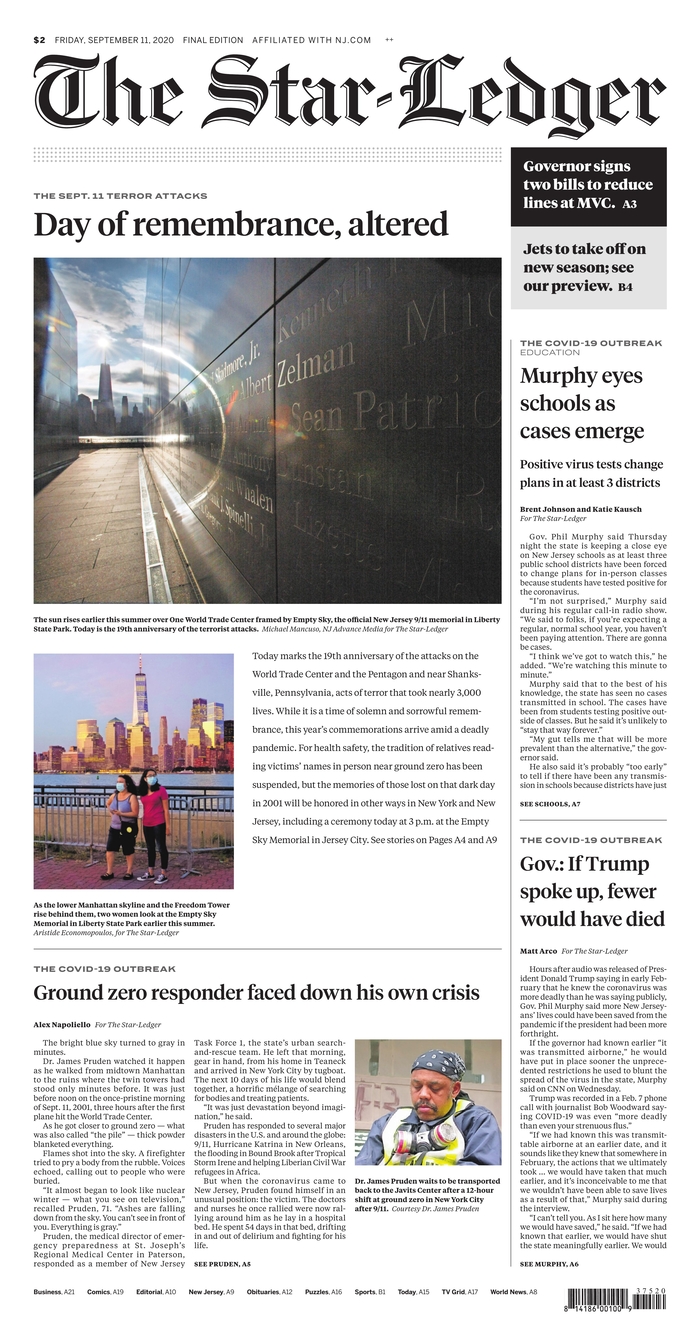The screen displays a webpage from the Star Ledger, designed to resemble a traditional newspaper layout. At the top, the masthead features "The Star Ledger" in a bold, classic newspaper font. Below the masthead, the main headline reads "Day of Remembrance Altered" in large, black text.

Beneath the headline, a photograph depicts a memorial wall inscribed with names. Below this image, another photograph captures two girls standing together, with an urban skyline visible in the background. Adjacent to this, a portion of an article is visible, including some introductory text.

Further down the page, a headline reads "Ground Zero Responder Faces Own Crisis," accompanied by several paragraphs of text. To the right of this article, there is a photograph of a man with his eyes closed, wearing a bandana and a blue shirt.

On the far right side of the page, additional articles are listed: 
- "Jets to Take Off on New Season"
- "Murphy Eyes Schools as Cases Emerge"
- "Gov: If Trump Spoke Up, Fewer Would Have Died."

Each headline is accompanied by introductory text, maintaining the appearance of a traditional newspaper.